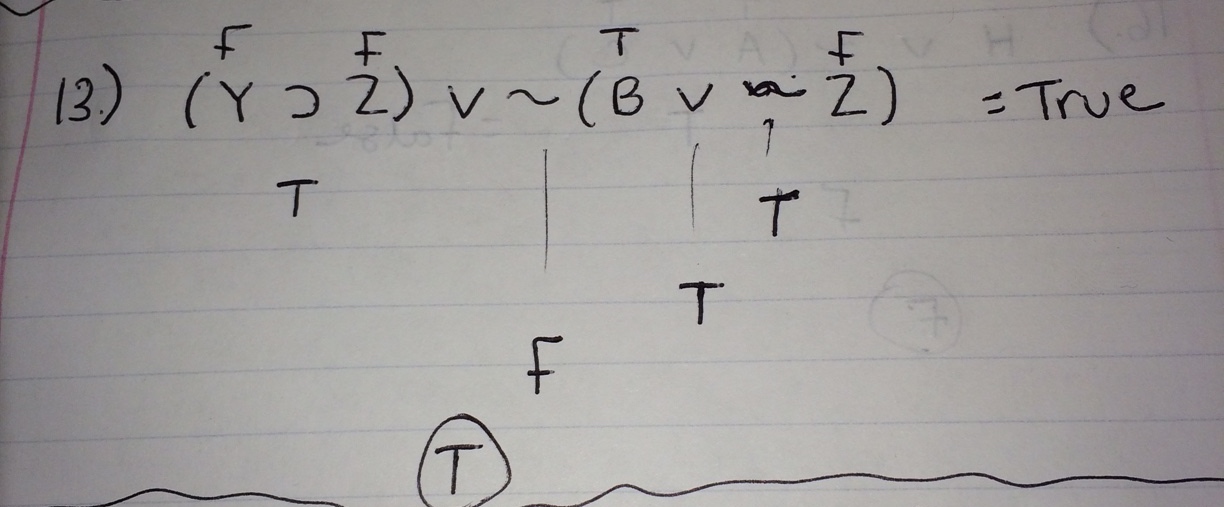This image showcases a handwritten mathematical equation on a white piece of lined notebook paper. The equation is complex and detailed, featuring various mathematical symbols and annotations. At the top, the notation begins with "13" followed by a period, then the expression "(Y ¬ C Z)". Above both the "Y" and "Z", the letter "F" is written. Adjacent to these parentheses, there is "V~", followed by another set of parentheses containing "(B V~ Z)". In this second set, "T" is written above the "B" and "F" above the "Z". The equation then states "= true".

Beneath the initial set of parentheses, the letter "T" is noted. A thin vertical line descends from the tilde (~) symbol to an "F". There is also a vertical line descending from the "V" in the second set of parentheses to a "T", and another line from the tilde (~) to a "T".

At the bottom of the page, there is a "T" encircled, flanked by long squiggly lines on both its left and right sides.

The dimensions of the image are notable—it is much wider than it is tall. There are no people, animals, or buildings present, maintaining the focus solely on the mathematical content.